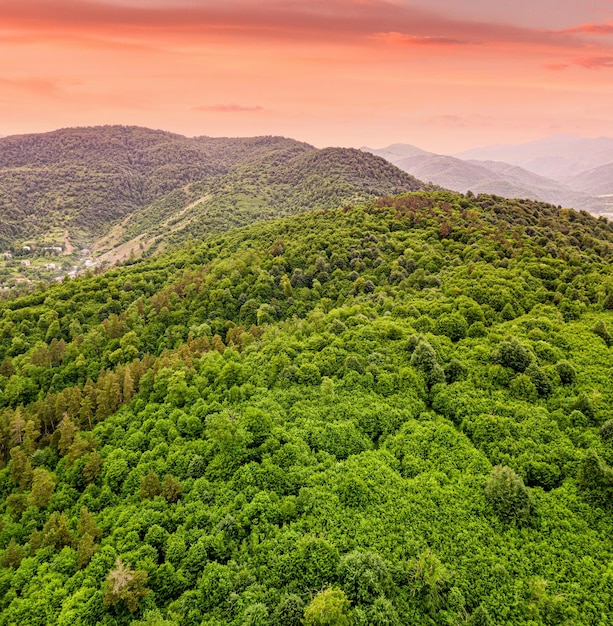The image captures an aerial view, possibly taken with a drone, overlooking a vast expanse of lush hills blanketed with green-leafed trees, stretching endlessly into the horizon. The terrain reveals valleys dotted with brown patches and dirt paths, suggesting trails suitable for hiking or mountain biking. In the background, a range of foggy, progressively blurred mountains emerges. The dramatic sky above is dominated by bright red, pinkish-red, and cotton candy clouds tinged with hues of orange, yellow, and purple, giving an impression of an impending sunset. The distant haze suggests the presence of a fire far off, with smoke drifting closer, adding to the surreal, atmospheric quality of the scene. On the left side, there appear to be some structures with white walls and roofs, faintly visible amidst the picturesque natural landscape.